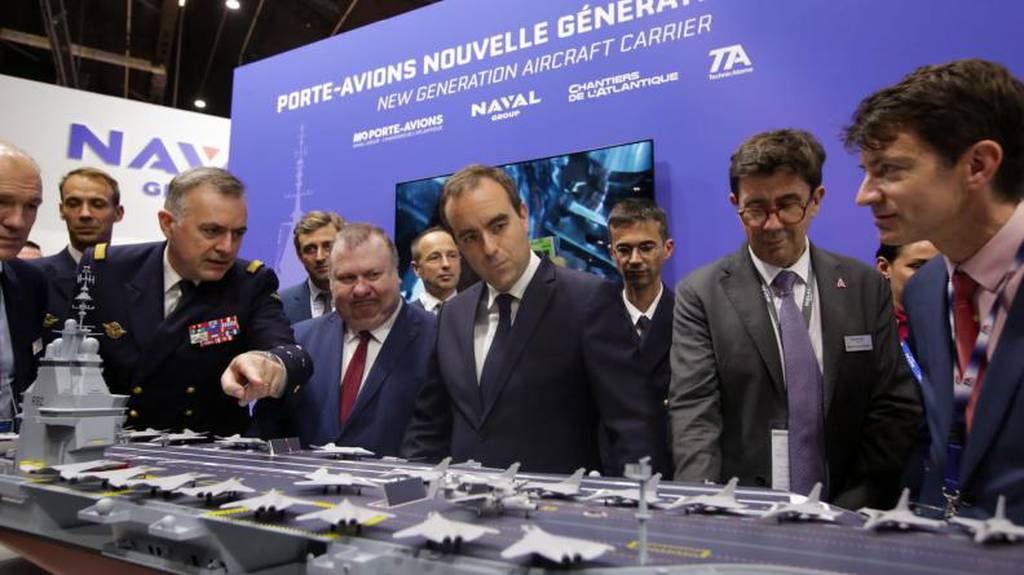The photograph depicts a group of approximately a dozen men gathered around a large, detailed model of an aircraft carrier. The men, mostly dressed in suits and ties, appear to be attentively observing the model while one man in a decorated military uniform with numerous badges is pointing towards it, seemingly explaining something. The model itself features hand-sized, gray fighter jets lined up on a runway that mimics a real aircraft carrier with black and white lines and a control tower at the end. In the background, a blue board with white fonts displays the text "Porte Avion Nouvelle Generale" and "New Generation Aircraft Carrier," alongside logos of three or four different businesses. Below the board, a television screen is also noticeable. The men seem engrossed by what they are seeing, suggesting a formal demonstration or briefing about the new generation aircraft carrier.